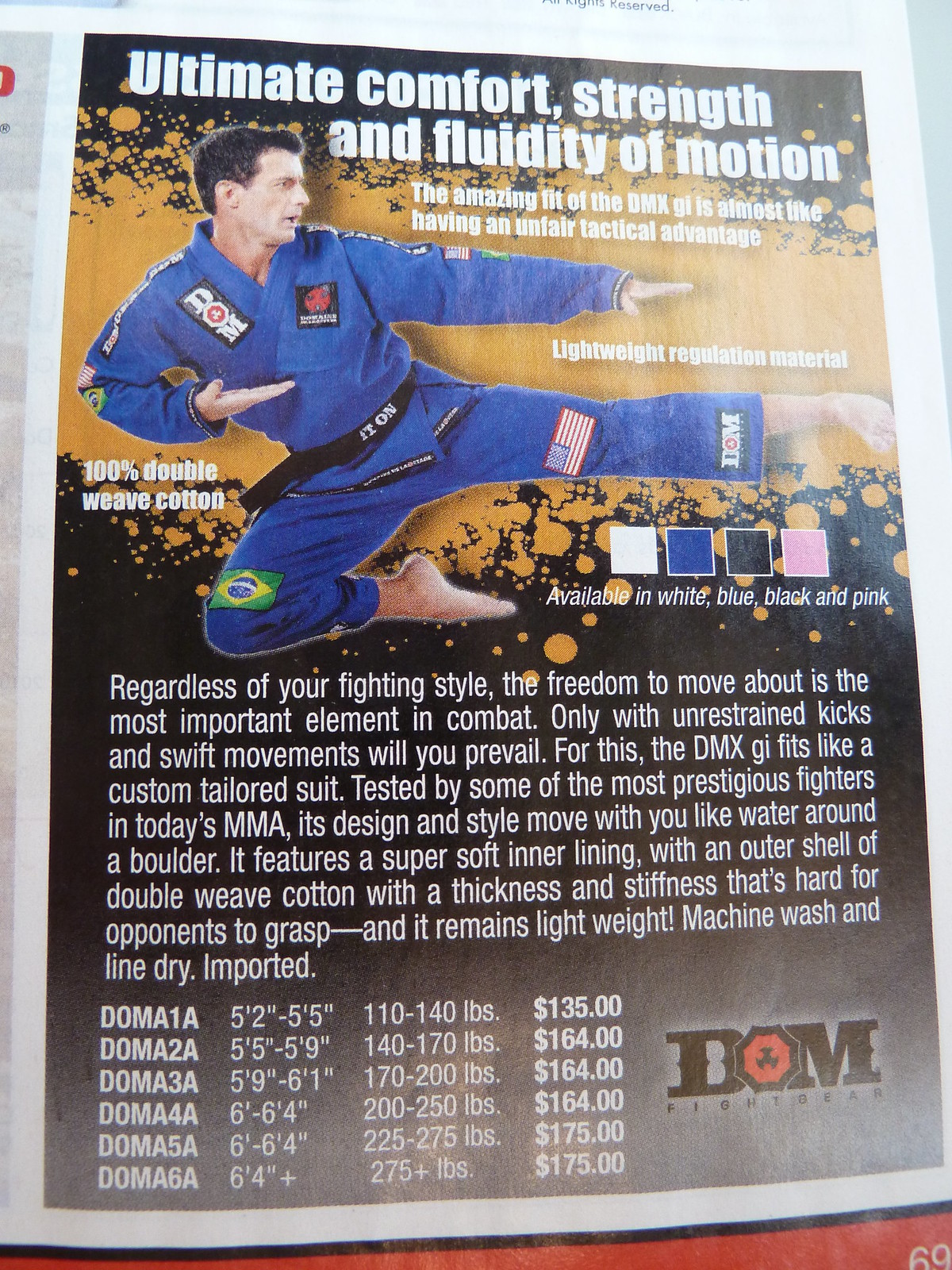The full-page advertisement showcases the "DMX Gi," designed for Mixed Martial Arts (MMA). At the top, bold white text proclaims the Gi's attributes: "Ultimate comfort, strength, and fluidity of motion." An image of a man in an acrobatic martial arts pose dominates the center. He wears a dark blue Gi adorned with numerous patches, including an American flag on his left knee and a Brazilian flag on his right. The man appears to be a focused Caucasian with brown hair, a black belt, and striking patches marked "D.O.M." He is depicted mid-air with a bent right leg and a pointed straight left leg, his arms dynamically positioned as if ready for combat.

On the left, additional text highlights the Gi's exceptional qualities: "100% double-weave cotton," "super soft inner lining," and "outer shell stiffness designed to be hard for opponents to grasp." The Gi promises "unrivaled freedom of movement," likened to "water flowing around a boulder." Tested by prestigious MMA fighters, the Gi is said to fit like a custom-tailored suit.

Below are detailed size and price charts. For example, the Gi is priced at $135 for heights 5'2" to 5'5" with weight classifications from 110-140 lbs, scaling up to $175 for heights exceeding 6' with higher weight brackets. The specs for these sizes are labeled as GOMA-A1A through GOMA-A6A. Finally, the bottom right corner features the "DOM Fight Gear" logo, emphasizing the brand's authenticity and quality.